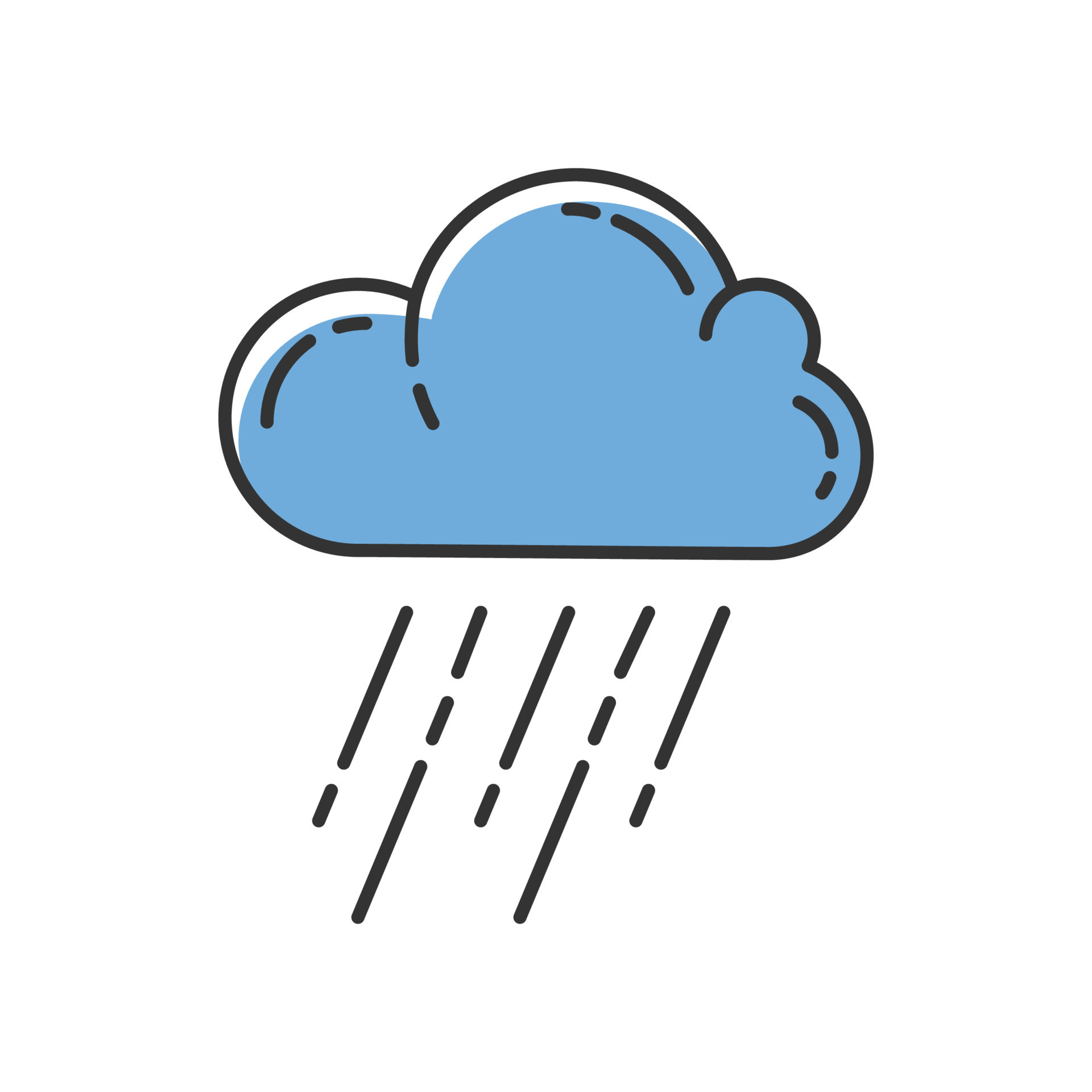This image features a simplistic, cartoon-style illustration of a rain cloud set against a completely white background. The cloud has a flat bottom with a pillowy, puffy top, resembling an ice cream scoop. It is filled with a soft blue color, highlighted with white at the edges, and is outlined in black. The cloud includes a couple of black circles and swirls, and a few small, black marks. Below the cloud, five diagonal, broken black lines angle to the left, each line adorned with either two or three black raindrops. This arrangement creates the impression of significant rainfall. The overall appearance is that of a typical rain cloud, characterized by its straightforward and unembellished design.